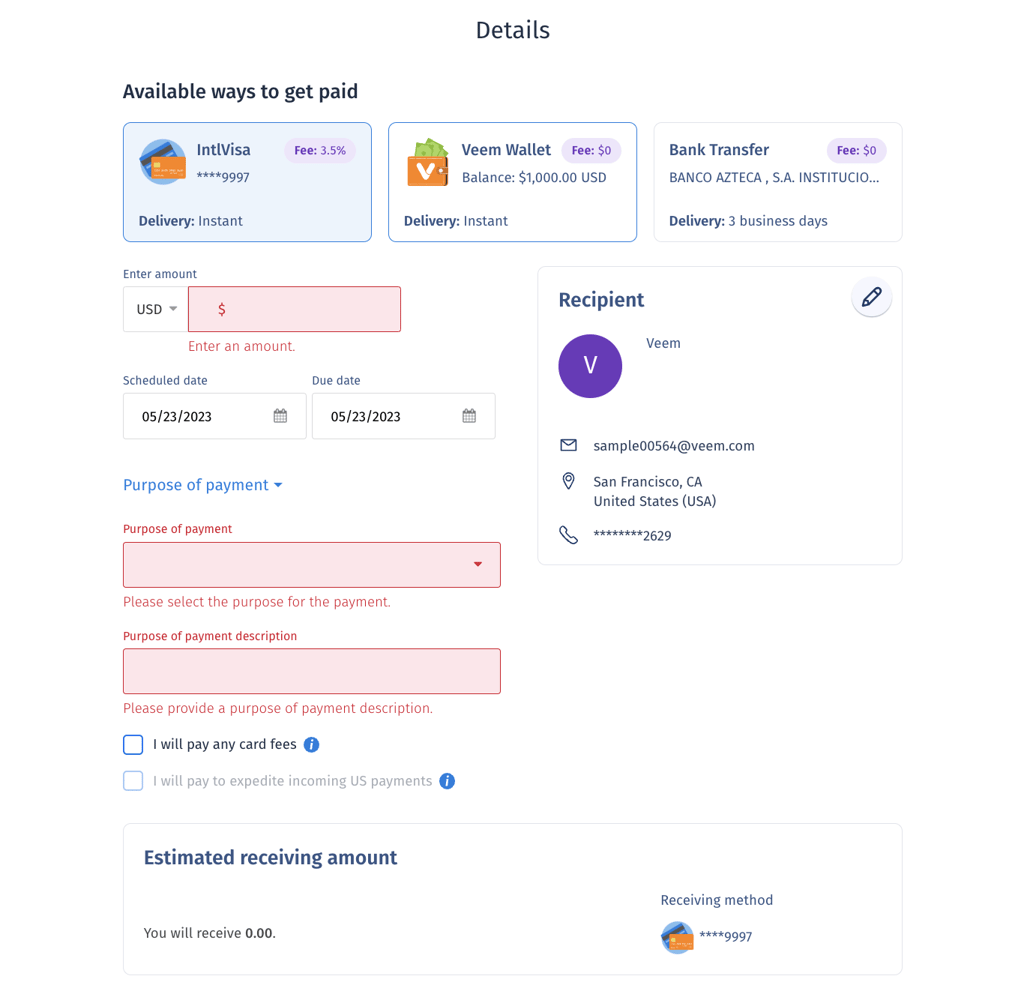Here is a cleaned-up and detailed caption for the image:

---

Screenshot of a finance app web page displaying payment options and details.

At the top, the header reads "Details." Below it, the section titled "Available Ways to Get Paid" features three rectangular icons, each representing a different payment method:

1. **Intel Visa**
    - **Fee:** 3.5%
    - **Rating:** Four stars
    - **Amount:** $99.97
    - **Delivery:** Instant
    - **Icon:** Two credit cards

2. **Veeam Wallet**
    - **Fee:** 0%
    - **Balance:** $1,000 USD
    - **Delivery:** Instant
    - **Icon:** Stack of money

3. **Bank Transfer**
    - **Institution:** Banco Azteca, S.A.
    - **Fee:** 0%
    - **Delivery:** Three business days
    - **Icon:** Bank building

Below these options, additional controls are available for processing a payment:

- **Enter an Amount:** User can input the desired amount for the transaction.
- **Schedule a Date and Due Date:** Options to set the transaction date and due date.
- **Purpose of Payment:** Two drop-down boxes for selecting the payment purpose and providing a description. Labels prompt users to choose options and describe the transaction.

At the bottom, two checkboxes offer additional payment handling options:
- **I will pay any credit card fees** (highlighted in blue and black)
- **I will pay to expedite incoming US payments**

Below these checkboxes, the section ends with a field labeled "Estimated Receiving Amount," where users can view the expected amount after deductions.

---

This version provides a clearer and more structured description, making it easier for readers to understand the contents and functionality of the app interface.